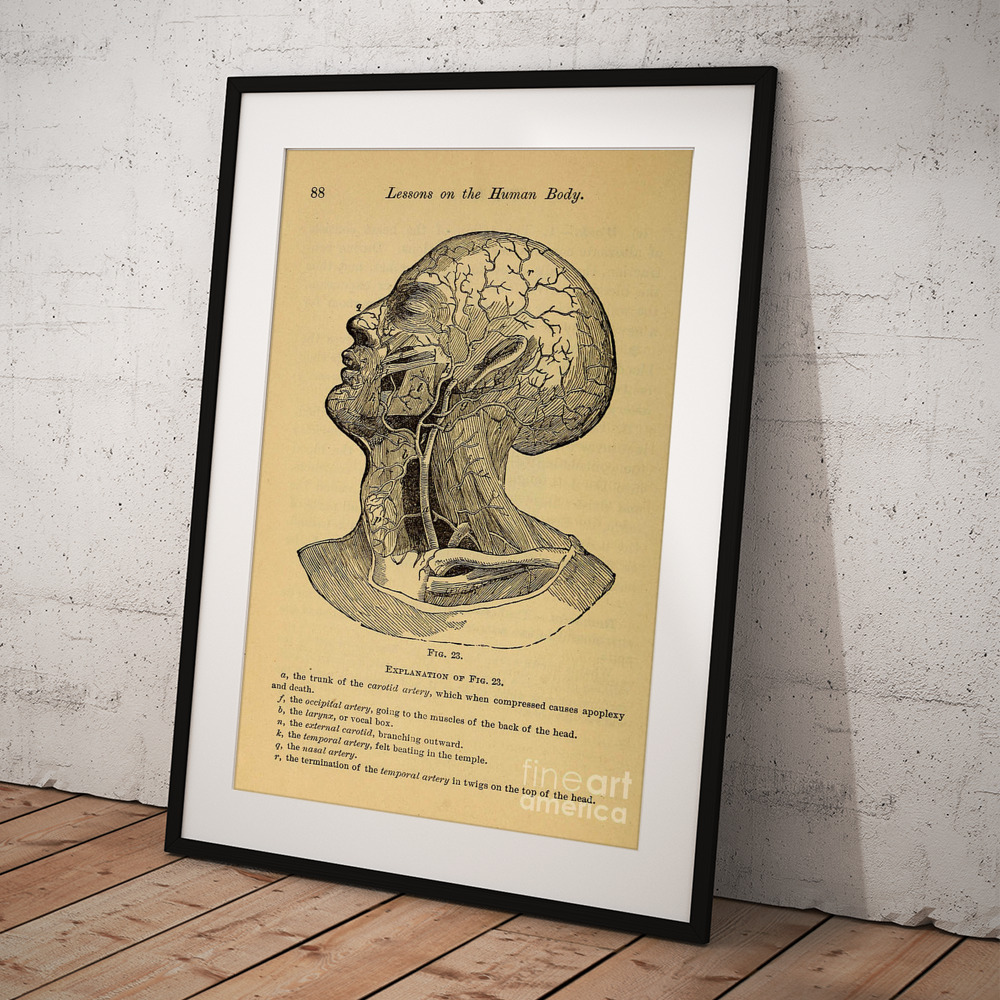This detailed photograph captures a framed medical illustration, reflecting the style of the late 1800s or early 1900s, hand-illustrated with pencil on yellowed paper. The drawing originates from a book, as indicated by "page 88" and the italicized title, "Lessons on the Human Body," at the top. The black frame with its white mat is propped against a white concrete wall on a wooden floor. The illustration depicts a human figure, eyes closed, facing left, with the skin removed to reveal intricate details of muscles, nerves, arteries, and veins extending from the head to the collarbone. The image corresponds to Figure 23, with a partially legible explanatory text beneath it. The print includes modern identification from Fine Art America at the bottom right.